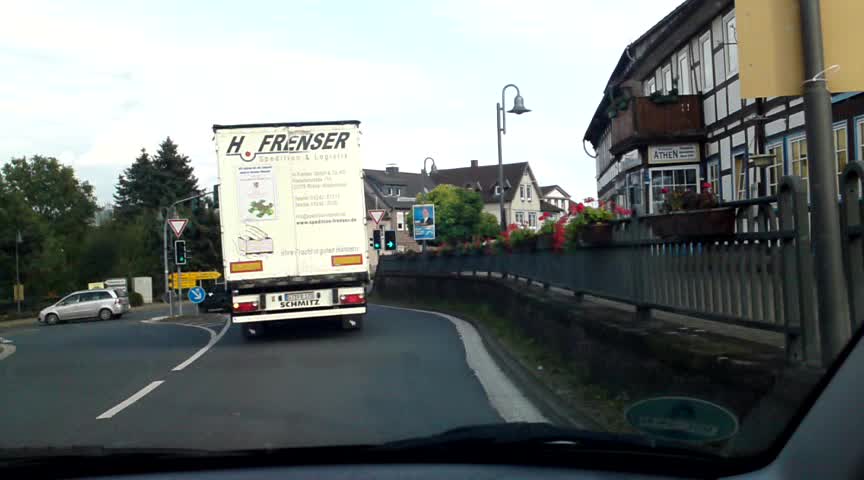In this photograph, a person is seen taking a picture of the rear end of a white truck, labeled "H. Forenser," parked on a street next to a multi-story building. The building, possibly a restaurant or shop, has numerous windows and a visible sign that reads "Athen." Adjacent to the building is a raised platform bordered by a metal fence adorned with flower pots, each brimming with vibrant blossoms that add a splash of color to the scene. A light post stands close to the fence, enhancing the quaint, urban street atmosphere.